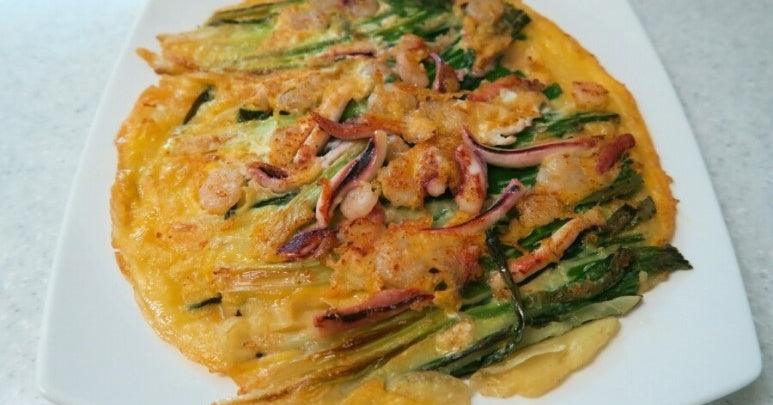The image depicts a round Korean seafood pancake, known as pajeon, elegantly presented on a square-shaped white plate. The plate rests on an off-white countertop, adding a clean and simple backdrop. The pancake itself showcases a vibrant array of ingredients: golden-yellow melted cheese dominates the surface, interspersed with visible pieces of octopus or squid legs, particularly towards the center-right. Cooked shrimp, displaying a pale pink-orange hue, are scattered across the pancake, with a notable concentration on the left side. Long, green asparagus spears are particularly prominent at the top and bottom of the pancake, adding a fresh element to the dish. The overall presentation suggests a homemade, ethnic delicacy, rich in color and textures, blending seafood with vegetables harmoniously.